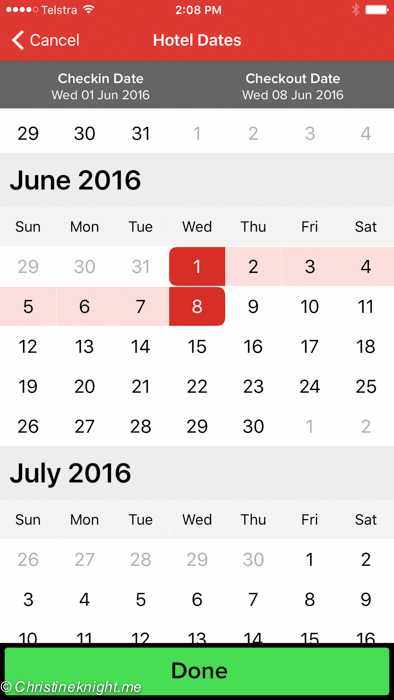The image displays the screen of a cell phone with various interface elements. At the top of the screen, the status bar shows the text "TELSTRA," along with icons for phone signal and Wi-Fi connectivity. The time reads 2:08 PM, and there is a full battery icon, all displayed in white font.

Below the status bar, there are two colored horizontal bars: the top bar is red, and the one beneath it is dark gray with white font. The text displayed on the gray bar reads "Check-in date: Wednesday, 1 June 2016" and "Check-out date: Wednesday, 8 June 2016."

The main section of the screen features a calendar for June 2016. The dates corresponding to the check-in and check-out are highlighted in red. A pink band stretches between these dates, indicating the duration of the stay. The numbers for these highlighted dates are white on a red and black background for the pink band. The rest of the calendar dates are displayed in black font on a white background.

The top of the calendar displays the month and days of the week ("June 2016" and "Sunday, Monday, Tuesday, Wednesday, Thursday, Friday, Saturday") in black font on a gray background.

Below the June calendar, there is a similar display for July 2016. It follows the same color scheme, with gray for the month and day names, and white for the calendar dates.

At the bottom of the screen, there is a button labeled "Done."